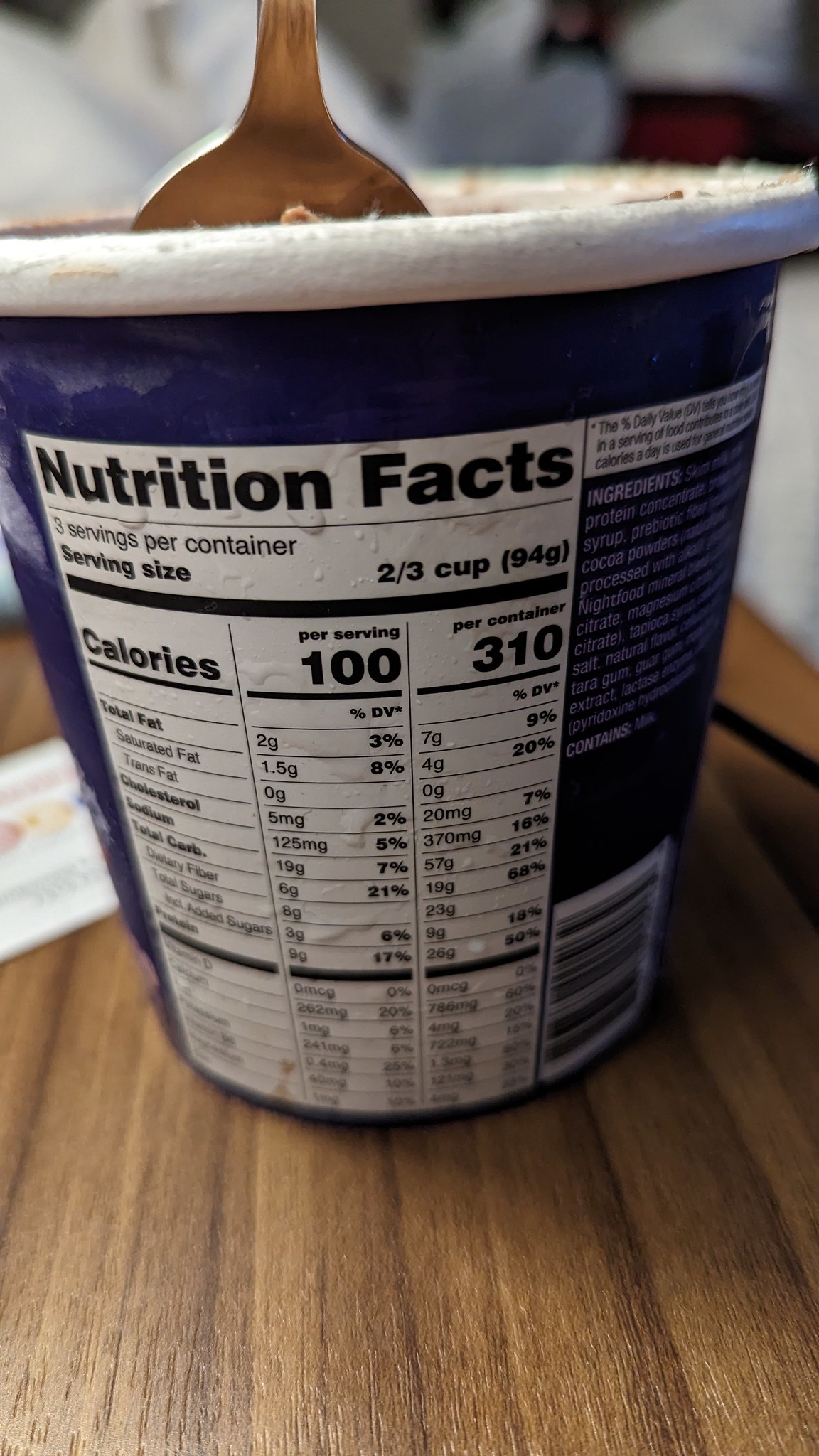The image features a pint of ice cream displayed prominently on a wooden table. The pint's dark blue container is adorned with a white label detailed with black text that highlights the nutritional facts. The label specifies that there are three servings per container, with calorie count and various nutritional values clearly listed. To the right of the nutritional facts, white text enumerates the ingredients, though most of this information is difficult to discern. A spoon is positioned upright in the ice cream, partially visible from the top of the container. The scene captures a moment of indulgence, emphasizing the essential details pertinent to those mindful of their dietary intake.